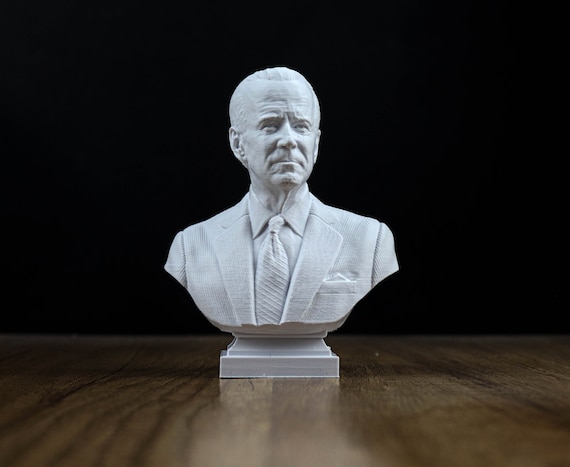The image features a meticulously sculpted bust of President Joe Biden, showcased against a black background. The bust, which appears to be all one piece, sits on a stone stand on a wooden table with swirling brown patterns. The sculpture captures Biden from just below his tie to the top of his head. His detailed features include a collared shirt, a striped tie, and a neatly folded napkin in his lapel pocket. Biden's expression is serious, highlighted by a furrowed brow and eyes looking straight ahead, with his mouth closed and slightly curved downwards. His thinning hair also contributes to the lifelike accuracy of the bust.